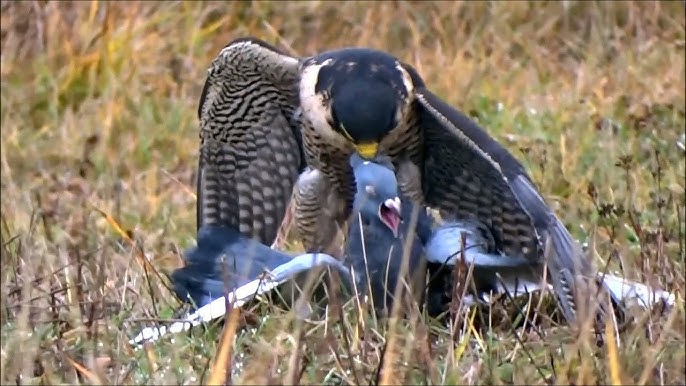In this detailed and dramatic wildlife scene, a large bird resembling a hawk or eagle grips a smaller bird in a brutal altercation. The imposing predator, distinguished by its black head, yellow beak, and speckled wings with black, white, and gray markings, appears to be attacking or feeding on the smaller victim. The smaller bird, dark gray with blue undertones, lies pinned on the ground, its beak wide open in a silent scream, eyes tightly shut in distress. The background is a natural setting of tall, thin grass—some green, some brown and dead—creating a dry, field-like atmosphere. Both birds are positioned centrally in the image, facing towards the camera, capturing a moment of raw nature with no visible signs of blood from this angle.